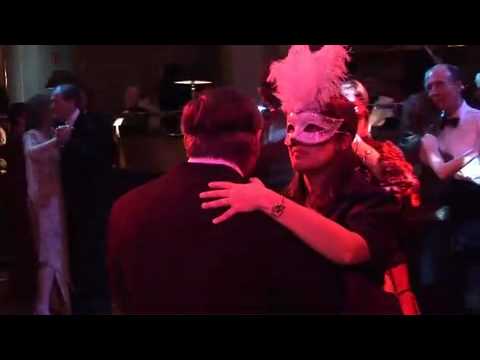In this evocative photograph, there's a central focus on a couple elegantly dancing amidst an opulent ballroom, illuminated by a red-tinted light that casts a warm, yet slightly mysterious glow over the scene. The man, seen from behind, wears a brown suit jacket and has short brown hair, giving a glimpse of what might be an elastic band indicating a mask. His partner, a woman, complements the scene with an intricately detailed masquerade mask adorned with large pink feathers that drape gracefully over her forehead. She is dressed in a formal brown or burgundy gown and accessorized with a bracelet on her wrist. They are enveloped in the ambiance of a masquerade ball, joined by several other couples in the background, all engaged in a slow, close dance. The room, dimly lit with a lamp visible in the background, features other elegantly dressed individuals, the men in suits and ties or bow ties, enhancing the formal and festive atmosphere. A lady in a white dress can also be glimpsed, adding to the diversity and grandeur of the gathering, as everyone revels in the enchantment of the masquerade.